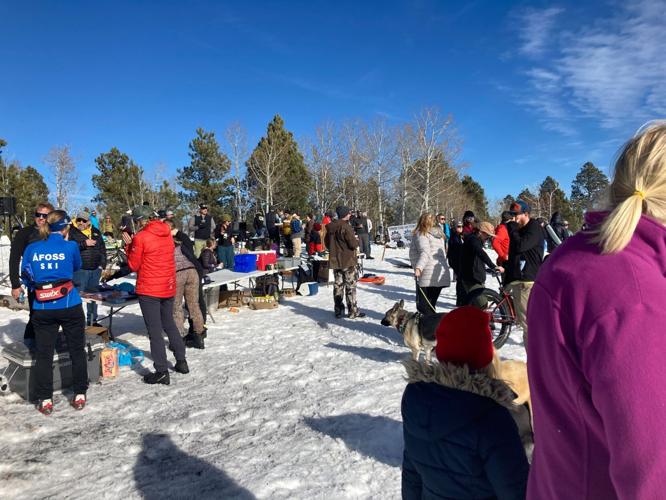This image captures a vibrant outdoor gathering at a ski area on a bright, clear winter day. The scene unfolds in a snowy meadow, not part of the ski slope, with dozens of people mingling around. The snow on the ground is heavily trafficked, appearing dirty and trampled. A row of tables with cooler chests filled with food or beverages stands slightly left of center. People dressed in cold weather gear, including a man in a ski jacket labeled "FOSS," are seen chatting and milling about. Nearby, a woman in a bulky white parka with a fur collar holds a Great Dane on a leash, and a mom with her daughter, wearing a purple jacket and a red ski cap respectively, stand with their back to the camera. Distinguishing individual features is challenging due to distance, but a few details stand out, like a person in a day-glo orange parka, likely a ski patrol member, and another with a bandana or headband covering their ears. The horizon is jagged with a mix of barren aspen trees and tall evergreen pines, and the sky is a deep, almost cloudless blue, except for some wispy clouds in the upper right-hand corner. The overall atmosphere is lively and picturesque against the pristine, alluring winter sky.